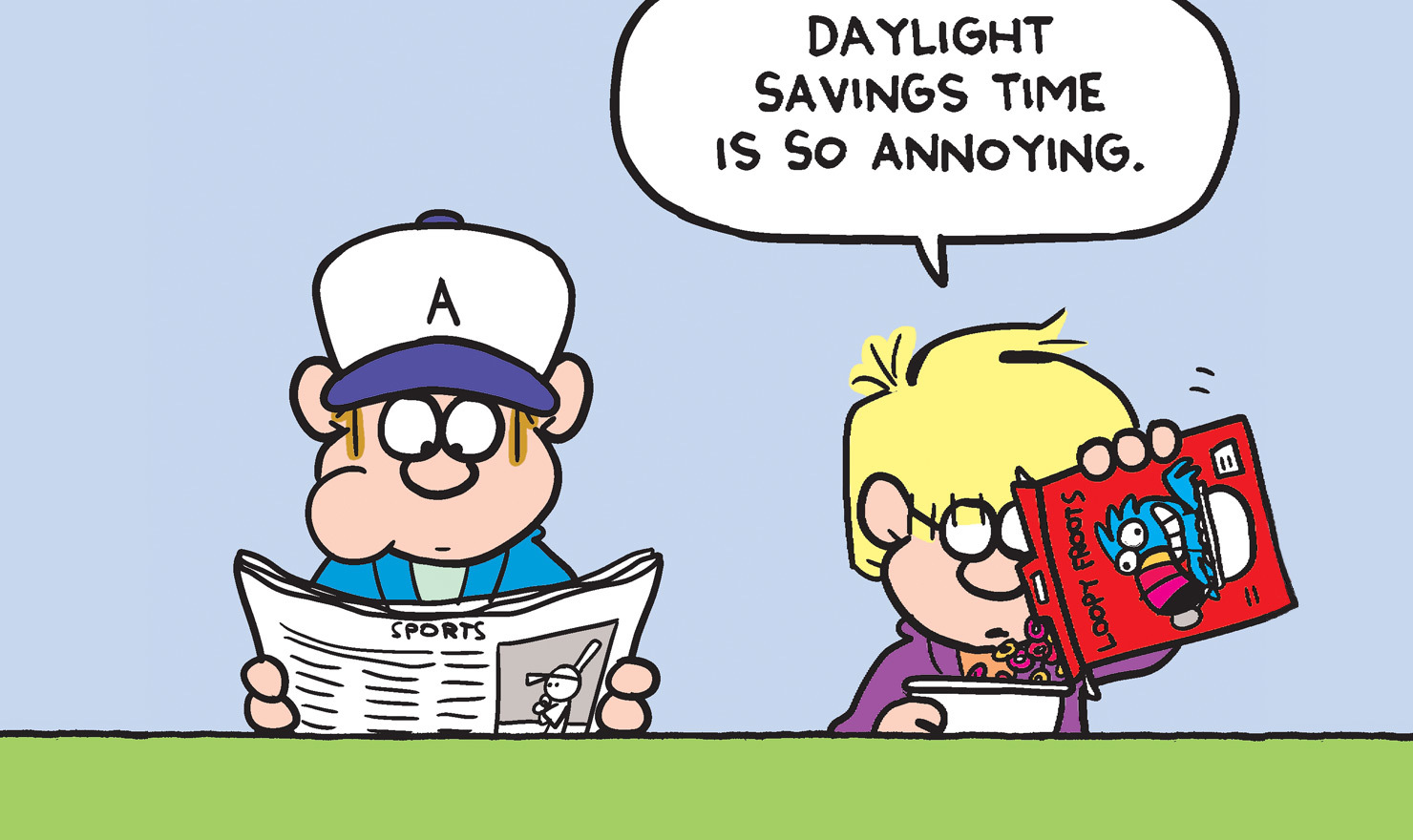In a rectangular cartoon, depicted in vibrant colors of green, blue, yellow, red, purple, white, and brown, two boys sit at a green table against a light blue background. The boy on the left, wearing a white baseball cap with a blue brim and the letter 'A,' chews gum and reads the sports section of a newspaper. He is dressed in a bright blue coat over a green shirt. His cheek is noticeably protruded. The boy on the right, with blonde hair and eyeglasses, dons a purple sweater and is pouring "Loopy Fruits" cereal from a red box into a white bowl. The cereal box features a toucan-like character and spells 'fruits' as 'F-R-O-O-T-S.' Above the boy pouring cereal, a speech balloon displays the phrase, “Daylight Savings Time is so annoying.”